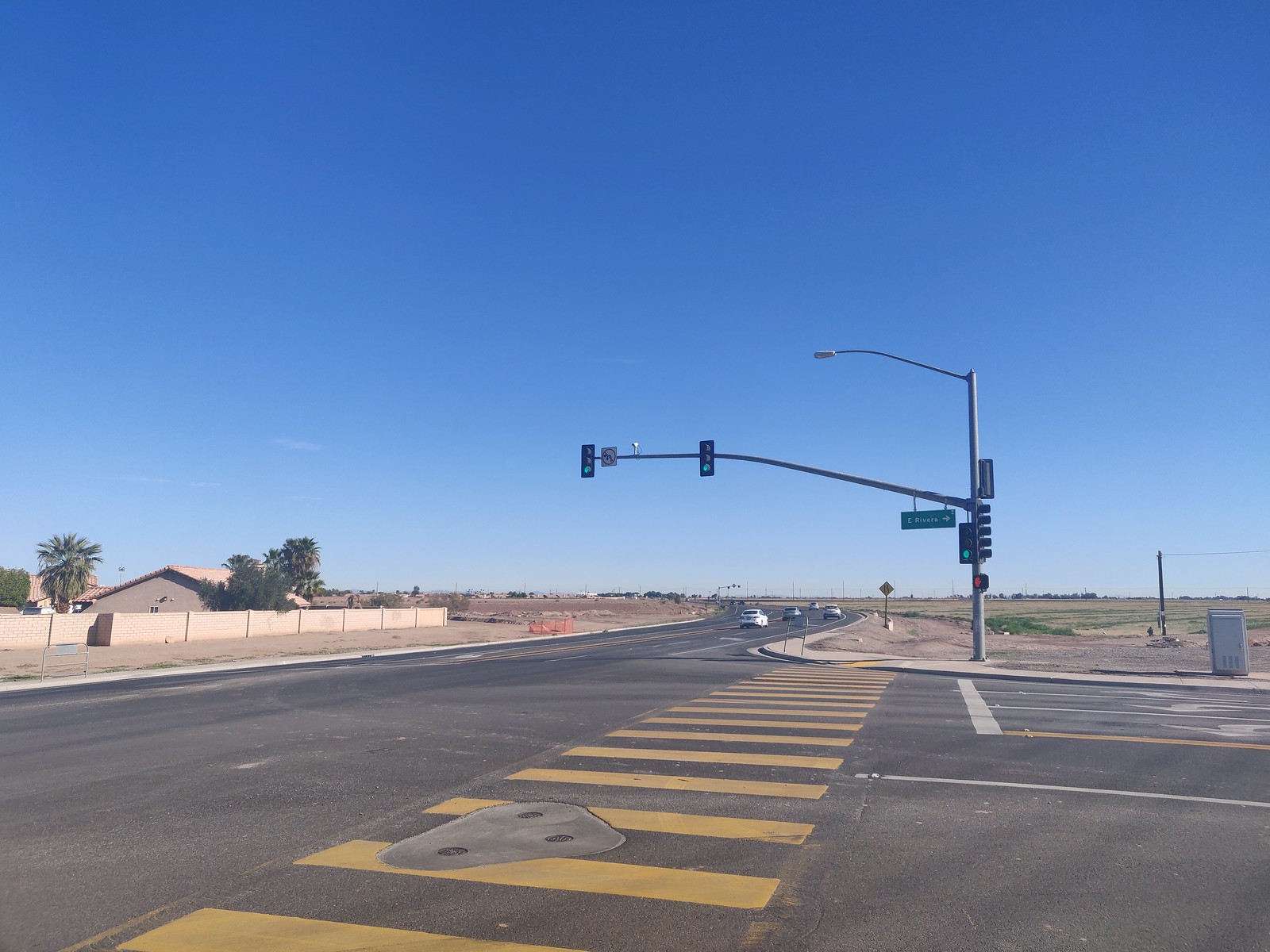The image captures a color photograph of a sprawling highway intersection set in a flat, dry, rural area, possibly in California, given the presence of several palm trees and the arid landscape. The top half of the photo is dominated by a cloudless, vivid blue sky, interrupted only by a streetlamp extending into the frame. 

On the left side of the image, a low wall encloses what appears to be a house or possibly a business, sitting close to the highway due to its low, peaked roof that resembles a residential structure. The wall could be made of yellow or white bricks, or possibly wood panels. Adjacent to this building are a few palm trees and other miscellaneous trees that add a touch of greenery to the otherwise sparse environment.

The highway itself, constructed from asphalt, appears to be a major road with four lanes. In the foreground, a yellow crosswalk featuring prominent yellow bars is visible, signifying pedestrian access at the lengthy intersection. This area also includes a concrete patch embedded within the road, containing three manhole covers. An adjacent large road with at least five lanes – including two left-turn lanes and a right-turn lane – converges from the right side of the photo.

Sidewalks flank both roads, running along the intersection and partially up the main highway, accommodating pedestrian movement. A few cars are seen traveling on the main road. 

A streetlamp mounted on a tall pole extends a long arm across the intersection, supporting two traffic lights, both displaying green signals. One of these lights also carries a no-left-turn sign indicated by a left-pointing black arrow contained within a red circle. Near the base of the arm, tied to the pole, hangs an indecipherable green road sign. Additional traffic lights, including a pedestrian signal box flashing a red hand, are mounted further down the pole, guiding traffic from the approaching secondary street.

The land stretching beyond the intersection is distinctly flat, boasting a horizon sprinkled with brownish grasses and a distant row of trees, reinforcing the rural characteristic of the scene.